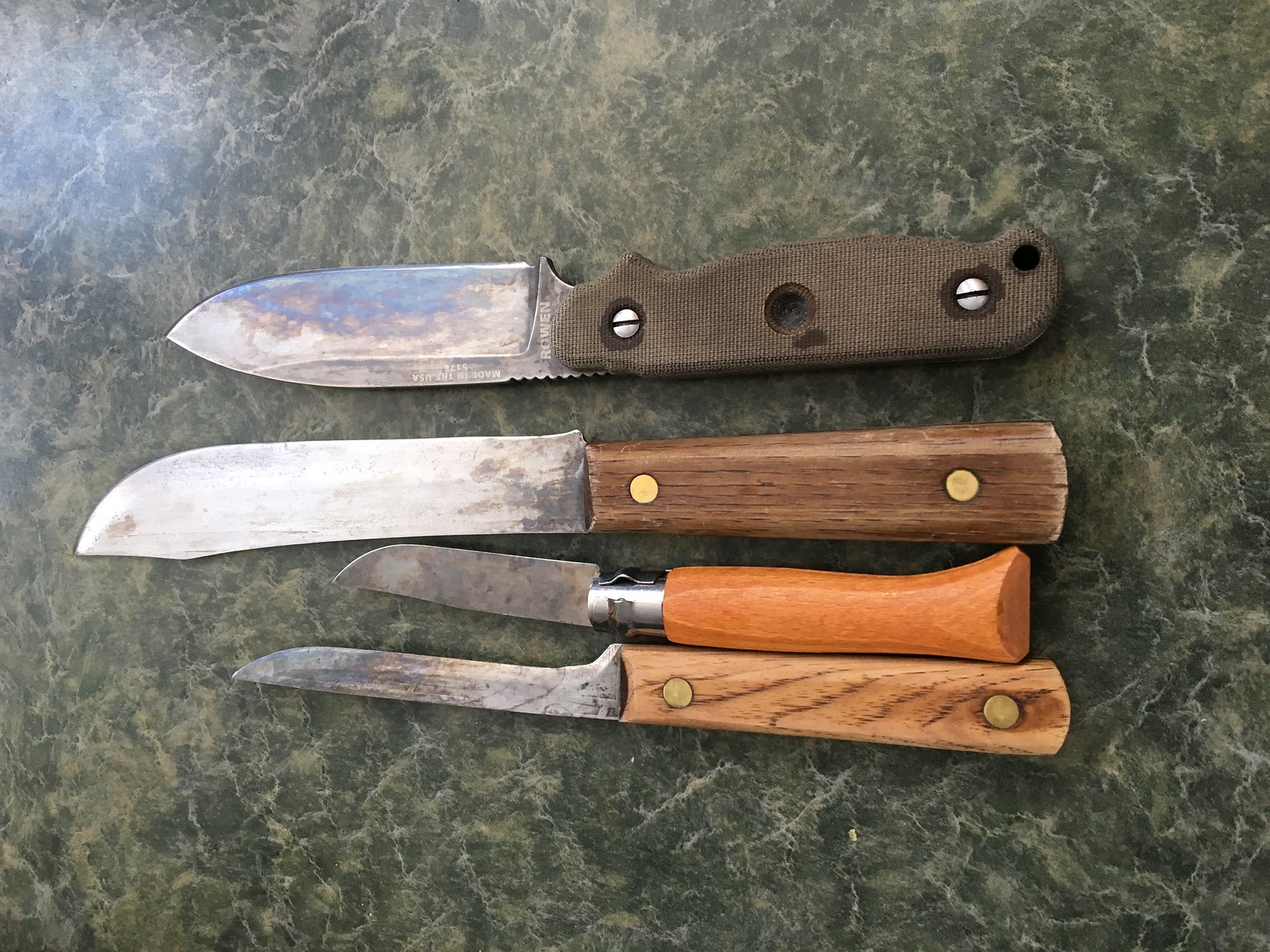The image is a close-up, aerial photograph featuring four aged and rusted kitchen knives laid horizontally on a dark green and black marble-like countertop. The lowest knife is a smaller steak knife with a light wooden handle and gold screws, displaying obvious signs of wear. The second knife above has a rounded, golden-brown wooden handle and a short metal blade, resembling a paring knife. The third knife is slightly larger, with a dark brown handle and a longer, visibly aged blade. The topmost knife appears to be a folding pocket knife with a rough grayish-brown handle, featuring a combination of smooth and serrated blade sections. All handles are in various shades of brown, suggesting extensive use and possible repurposing beyond typical kitchen tasks.